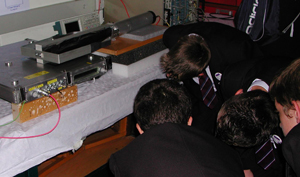The color photograph features several young boys, likely school-aged, dressed in matching black blazers with badges on the left side, white collared shirts, and black neckties with diagonal white stripes. They have short hair and are grouped together, either huddling or standing side by side, examining a table draped with a white tablecloth. On the table, there are numerous pieces of electronic equipment, including many small metal boxes with dials and ports. One of the prominent metal boxes on the top has a bright red cable extending from it, which trails out of the frame. The boys appear to be intently focused on these mechanical devices, though the exact nature and purpose of the machines are unclear. The overall scene suggests an educational or demonstrative setting.